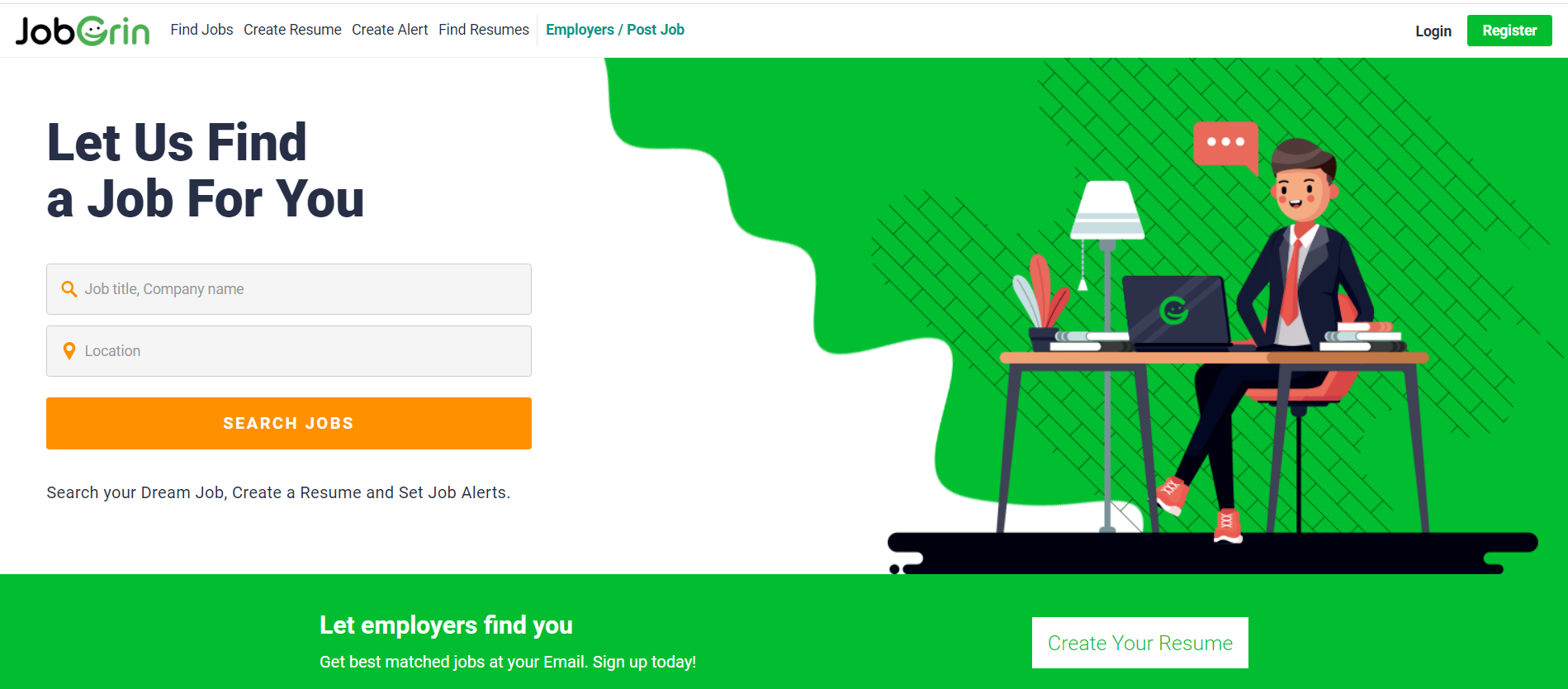**Detailed Caption:**

The image depicts a professional job search website's interface filled with various functionalities and vivid design elements to assist job seekers. At the top of the image, a banner features the headline "Job Grin." Below this headline, navigation options are listed, including "Find Jobs," "Create Resume," and "Create Alert." On the right side of the banner, user access options such as "Log In" and "Register" are displayed on a green bar, accompanied by the prompt "Let us find a job for you."

Directly below the banner, two input boxes allow users to specify "Your Job Title" and "Your Company Name and Location." Each input box is accompanied by an orange icon, enhancing their visual appeal. Adjacent to these input fields is an orange "Search Jobs" button, accompanied by the text "Search your dream job, create a resume, and set job alerts."

On the right side of the image, a professional illustration portrays a man wearing a suit with an orange tie and matching orange shoes. He is seated at a table with his laptop open, a table lamp, and some books placed to his left. The man's workspace is set against a vibrant background, with a black floor or platform beneath him and a green backdrop extending horizontally across the scene. 

Below the illustration, a green bar emphasizes the message "Let employers find you" and features a white button labeled "Create your resume." Additional small print appears underneath this prompt, providing further details or instructions for users.